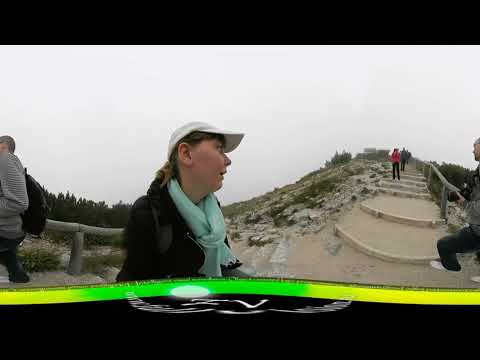In this color landscape photograph, bordered by black horizontal strips at the top and bottom, a panoramic filter combines two distinct images into one cohesive scene. The bottom strip features a narrow wavy band, transitioning from yellow to bright green with a moon-like emblem in the green section, alongside a design resembling a bird. Central to this composite image is a young lady in a dark jacket, light blue scarf, and white ball cap, her light brown hair pulled back as she looks to her right, seemingly engaged in conversation with an unseen person. She stands beside a wooden railing, and behind her, a man in a gray jacket faces left. The scene transitions to a stairway climbing a hillside with sandy platforms, rocks, greenery, and another wooden railing on the right. Several people are seen ascending the stairs towards the hilltop under a sky dotted with white clouds. The hiker's attire varies from pink and black to gray, emphasizing the crowded yet scenic path they traverse. The panoramic filter elegantly merges the two perspectives, capturing the essence of both the conversation and the bustling, picturesque trail.